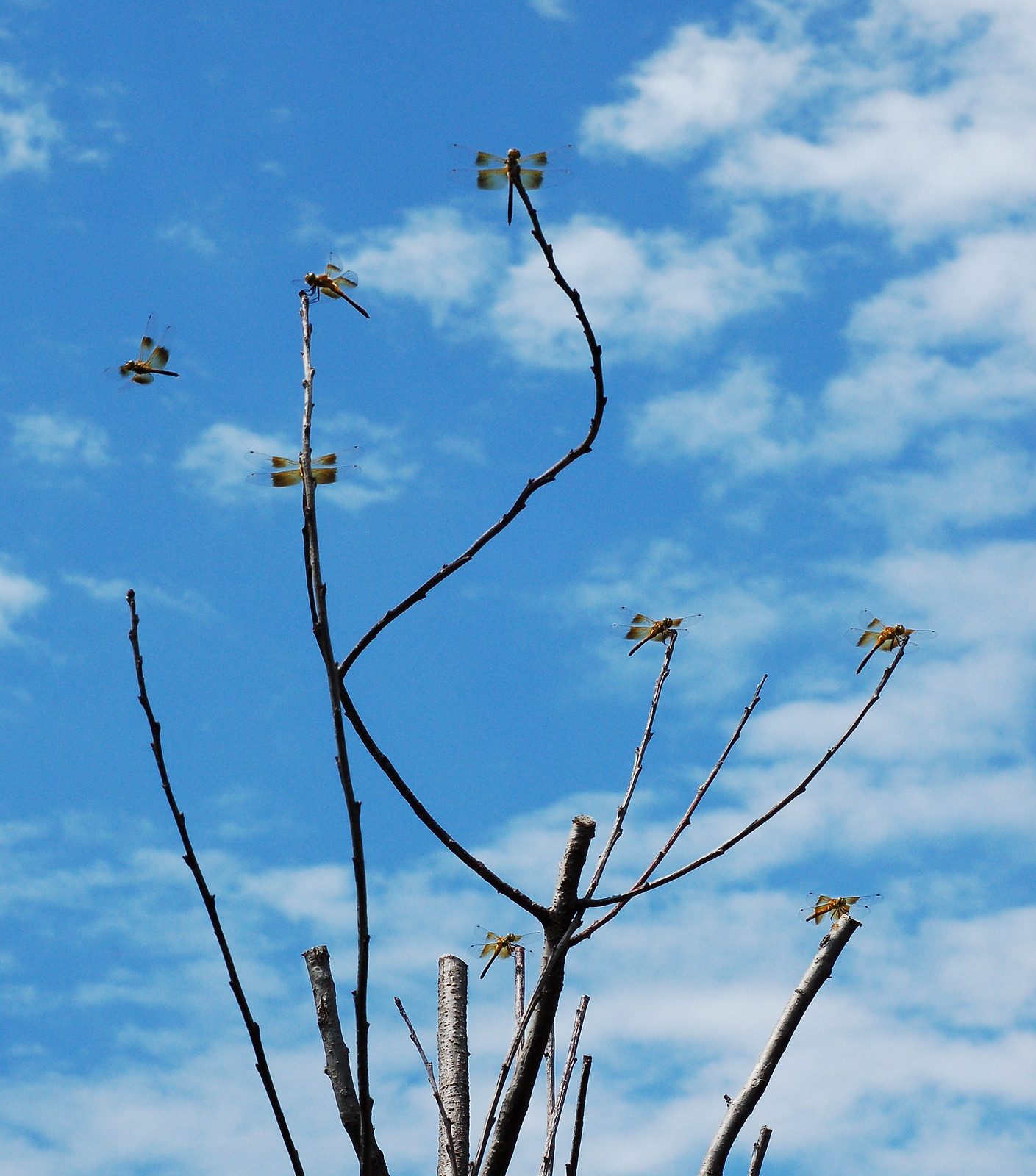In this outdoor photograph, a vast blue sky dotted with fluffy, partly cloudy patches takes up the entire background, suggesting a bright midday. Below the sky, the top of a leafless tree with thin, trimmed branches extends upward, each branch adorned with several twiggy offshoots. Perched prominently on these twigs are eight dragonflies, their bodies glistening with hues of green, red, and yellow. Seven dragonflies rest, delicately balancing on the twig tips, while one dragonfly is captured in mid-flight to the left, either taking off or preparing to land. The scene vividly captures the serene moment, blending the vibrant sky and nature's intricate details.